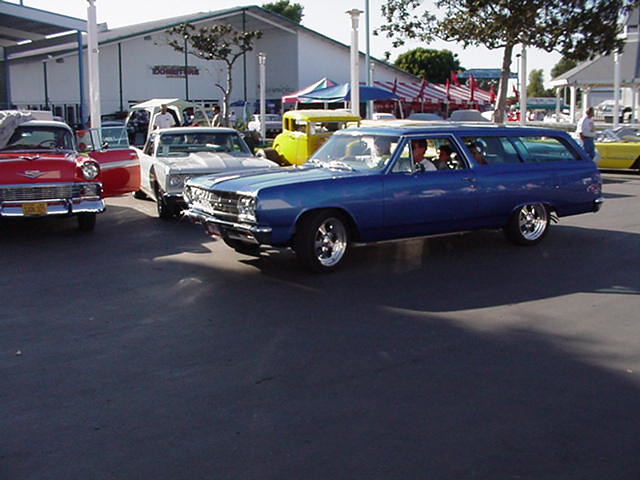This photograph captures a vibrant scene at what appears to be a classic car show held in a parking lot, possibly from recent years despite the vintage feel. The focal point of the image is a pristine, shiny blue late-model Volkswagen station wagon driving from right to left. The car’s deep chrome and beefy rims accentuate its well-maintained appearance. Inside the station wagon, there’s a man seated in the front, with another person, likely a woman or another man, next to him, and possibly children in the back seats.

The parking lot is dotted with an array of old cars, including a red and white car facing the camera, which could be an old Ford or Edsel, and a white vehicle that might be a Ranchero or old El Camino, featuring a distinct raised section on its hood. Additionally, a yellow car that resembles a Woody from the 50s stands out among the parked automobiles.

Surrounding the lot are several pop-up tents, including a prominent red and white striped one, a red, white, and green tent, and a solid blue tent, suggesting the bustling atmosphere of an event. Various people can be seen walking around, admiring the classic cars. The backdrop includes a large, pitched-roof building, a warehouse-type structure, and dense green trees with light brown trunks. The pavement is gray, and the overcast sky casts shadows from the nearby buildings and trees, adding to the nostalgic ambiance of the scene.